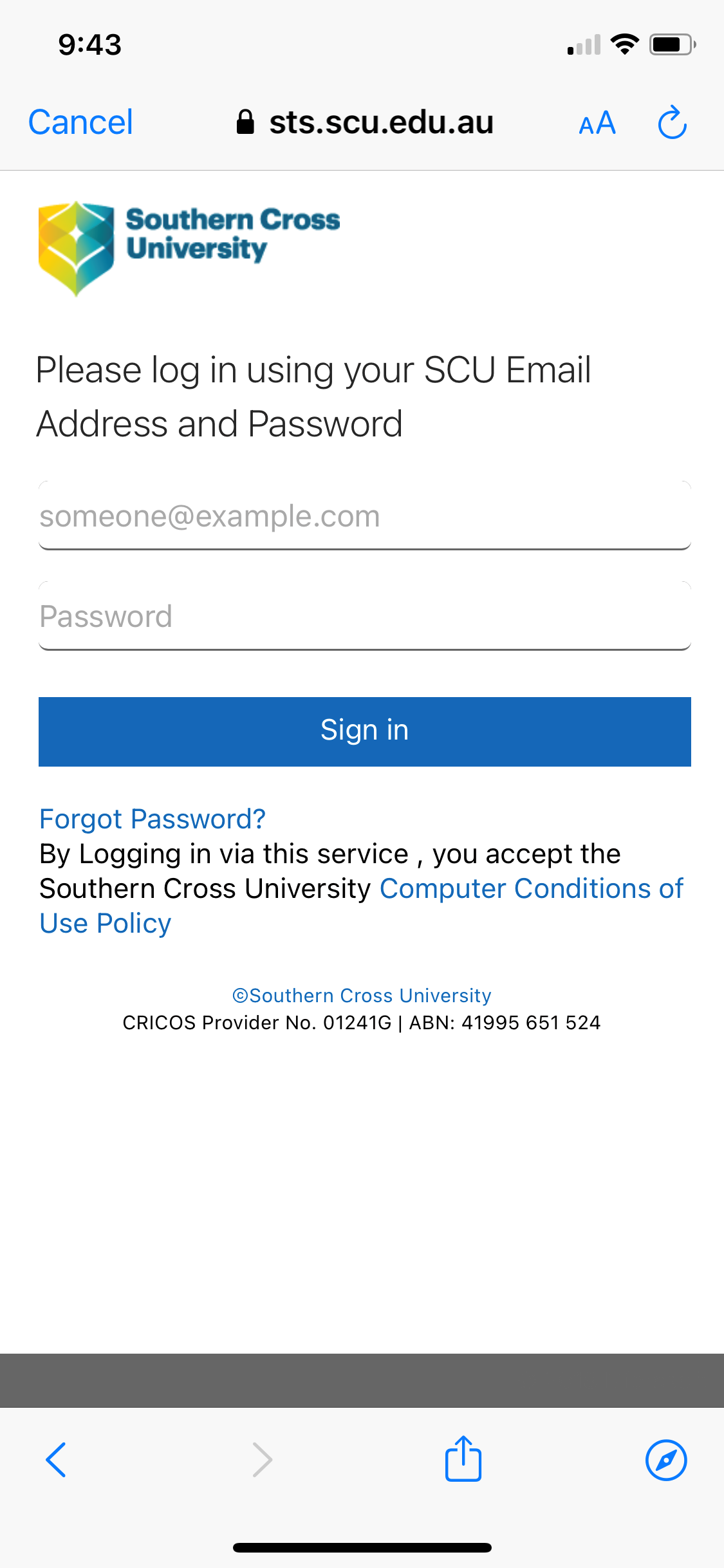A detailed caption for the image described:

"The image captured from a cell phone screen shows the login page for Southern Cross University’s online portal (sts.scu.edu.au). The top of the screen features the university logo with swirls of green, orange, yellow, and teal. Adjacent to the logo is a navigation bar with a blue 'Cancel' button, a small capital 'A' next to a large capital 'A’ for text resizing, and a refresh button. Below, the user is prompted to 'Please log in using your SCU email address and password.' Two input fields are visible: one for the email address, pre-filled with 'someone@example.com,' and another for the password. Beneath these fields is a blue rectangular 'Sign In' button in white text. At the bottom, there is a 'Forgot Password?' link in blue text with a question mark icon. Additionally, a disclaimer informs users that 'by logging in via the service you accept the Southern Cross University computer conditions of use policy.' The lower part of the screen displays a blank white area followed by a light gray rectangle containing clickable icons."